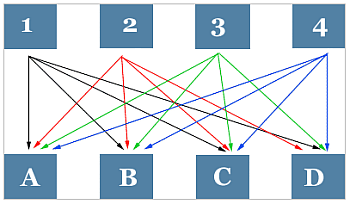The image is a detailed color illustration of a flowchart, presented on a white, rectangular background bordered by a thin gray line. At the top of the rectangle, arranged horizontally, are four slate blue squares, each containing a white number (1, 2, 3, and 4) in a Times New Roman style font. Between each blue square is a blank space approximately the same height as the square but not as wide.

Similarly, at the bottom of the rectangle are four blue squares with white letters (A, B, C, D) also in a Times New Roman style font, placed in a row and separated by blank spaces similar to those at the top.

A network of arrows connects the numbered squares at the top to the lettered squares at the bottom. Specifically:
- Black thin arrows lead from the square labeled "1" to each of the lettered squares (A, B, C, D).
- Red thin arrows extend from the square labeled "2" to the squares labeled A, B, C, and D.
- Green thin arrows originate from the square labeled "3" and point to A, B, C, and D.
- Blue thin arrows connect the square labeled "4" to each of the lettered squares (A, B, C, D).

Notably, there are no arrows connecting the numbered squares to each other, nor are there arrows between the lettered squares. The flowchart thus illustrates a one-way connection from each number to each of the letters.